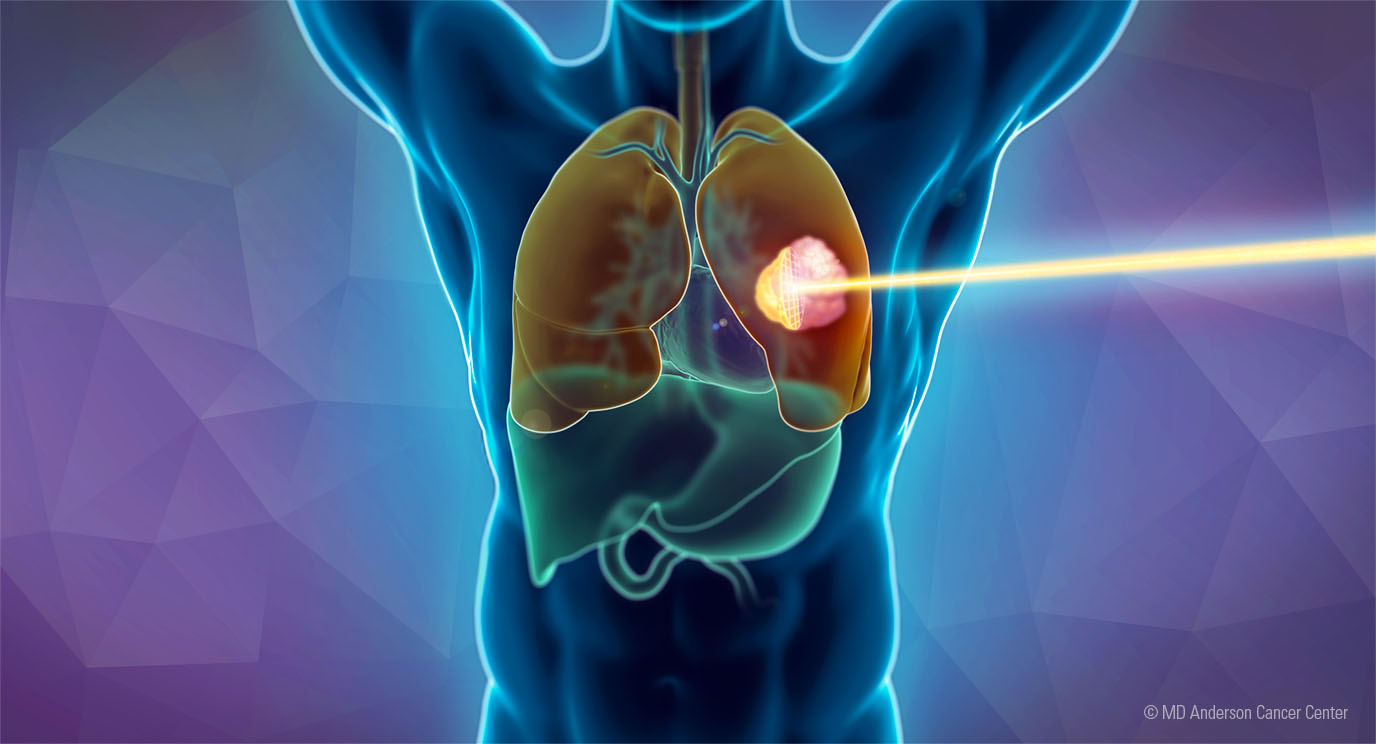The detailed illustration depicts a human body, specifically a man's torso, seen from below the chin to just above the hips, with his hands raised. The body is outlined in dark blue against a background that transitions from dark blue to purple with geometric patterns. The internal anatomy is visible, including brown lungs, the esophagus, stomach, liver (in green), and blood vessels. A striking feature is a bright, yellow-white laser beam with a blue outline emanating from the right side of the image, targeting an object or growth in the right lung (the left lung from the man's perspective), causing a noticeable impact. The image is approximately six inches wide and three inches high, and in the lower right corner, difficult-to-read white text says "Copyright MD Anderson Cancer Center."